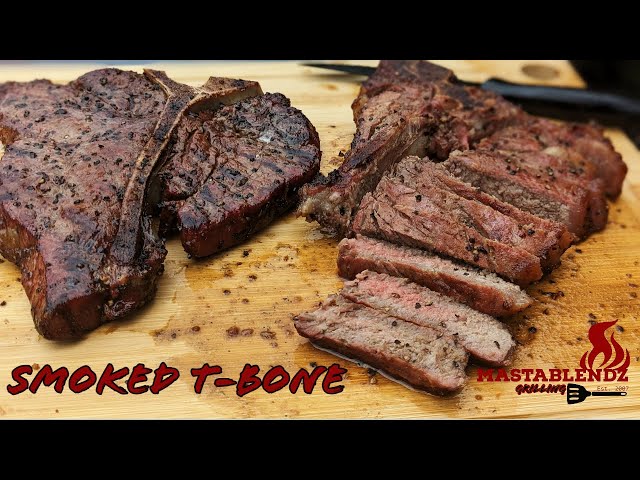This horizontal advertisement image features a tantalizing T-bone steak presented on a rustic wooden cutting board. Prominently, there is a perfectly smoked T-bone steak positioned on the left side, showcasing its juicy, well-seasoned exterior. To its right, the steak has been expertly sliced into long, appetizing pieces, revealing the succulent, tender interior. In the upper right corner of the cutting board, a steak knife is slightly blurred, hinting at the preparation process. The entire cutting board is centrally framed within the photograph, which is bordered by black bars at the top and bottom, directing the viewer's focus to the main subject and accompanying text. Centered at the bottom of the cutting board, bold red letters spell out "Smoked T-Bone." Adjacent to this text, on the right side, is the "Master Blends" logo, featuring a spatula and stylized red flames, signifying the brand behind the exquisite seasoning used on the steak.